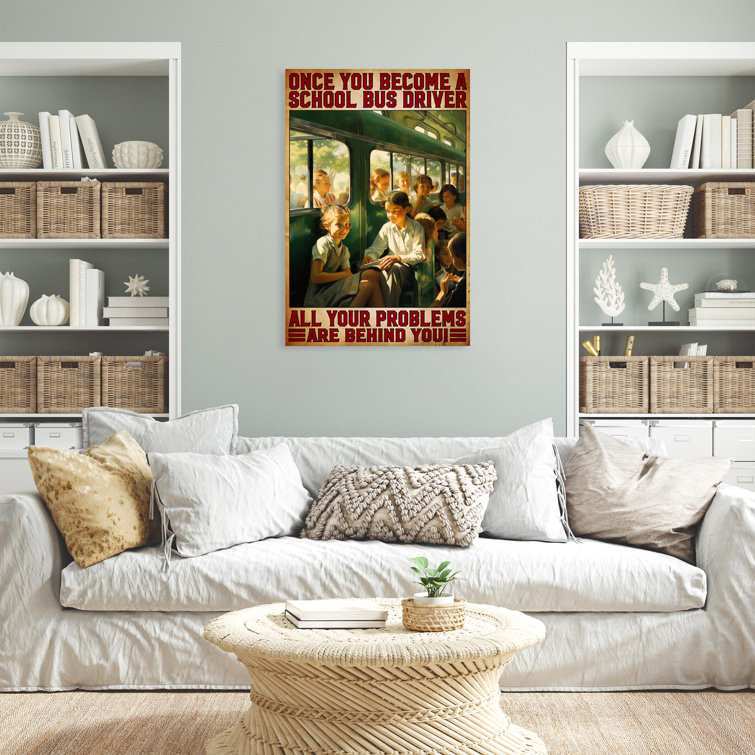The image depicts a cozy living room with gray walls and a wooden floor, highlighted by a satirical poster at the center. This prominent poster, mounted above a low-rise white sofa with wrinkled loose fabric, humorously proclaims, "Once you become a school bus driver, all your problems are behind you," accompanied by illustrations of a greenish-brown bus filled with children. The sofa is adorned with six pillows in various shades of white and gray, with one striking pillow on the far left being yellow with brown spots. In front of the sofa, there's a small, round wicker coffee table bearing two books and a tabletop plant in a white planter. Flanking the poster, built-in white bookshelves house an eclectic mix of books, white ornate decorations, marine-themed items like starfish and coral objects, and an assortment of wicker baskets.